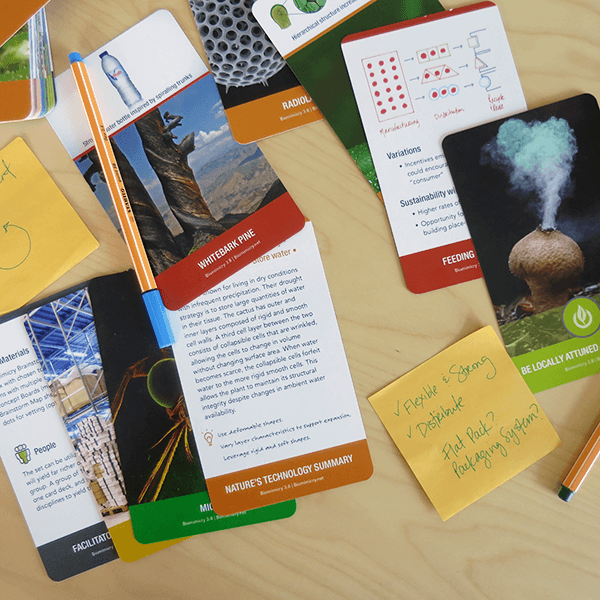In this image, we have a light brown desk scattered with various items, primarily centered around nine educational pamphlets, with some overlapping each other. Visible pamphlets include titles like "White Bark Pine," "Nature's Technology Summary," "Be Locally Attuned," and "Feeding." Some cards display images while others exhibit textual content, all seemingly educational and technology-focused. Surrounding the pamphlets are additional items: several blue-capped pens mistaken for pencils, an eraser-like object that lacks a clear point, and two sticky notes. One orange sticky note prominently features a checkmark, accompanied by the phrases "Flexible and Strong" and "Flat pack? Packing system?" A second yellow sticky note is partially visible on the opposite side of the arrangement. In the background, there is also a small stack of additional pamphlets, though their details remain obscured.